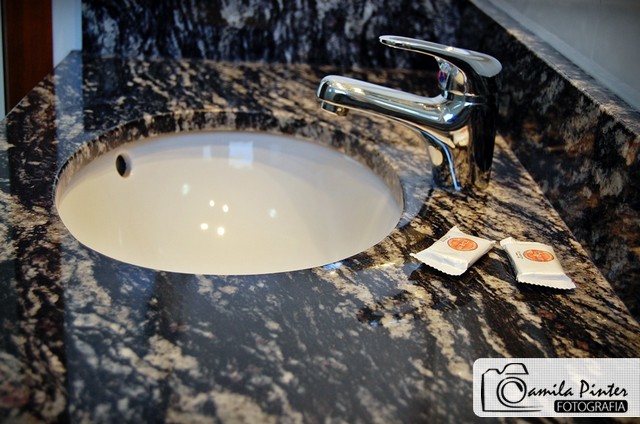The photograph is a meticulously composed product shot of a bathroom sink captured from an oblique angle, focusing on the right side. The sink's sleek, shiny metal faucet, with its elegant silver finish, rises from the upper right-hand quadrant of the image. It gracefully extends leftward, slightly angled upwards, accompanied by a handle aligned in the same direction.

The countertop is a dark granite surface, characterized by its striking irregular patterns of black interspersed with intricate veins of light tan. This natural stone serves as a luxurious base for the pristine, round, shiny white ceramic bowl of the sink.

Foregrounded in front of the faucet are two small white plastic packages, each adorned with a circular logo featuring shades of orange and red. The packaging, approximately an inch and a half long and an inch wide, appears neatly cut with a distinctive zigzag pattern on their ends. The text within the logo is somewhat blurry, rendering it unreadable at this resolution.

In the image's bottom right corner, a superimposed graphic watermark likely identifies the company behind the photograph. The design features a stylistic "C," followed by the words "Camellia Pinter," with "Photographia" beneath, set against a contrasting black background with white text. Adjacent to the text is a subtle camera outline, all framed on a clean white backdrop, enhancing the professional branding element of the image.